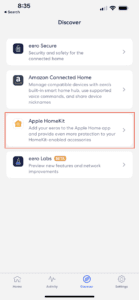A blurry snapshot taken on a cell phone captures an open application. Despite the unclear text, the black font is somewhat discernible. At the top left corner, the time reads 8:35, while the right side displays the battery charge indicator, Wi-Fi symbol, and a signal strength showing two illuminated bars. The top center of the app features the word "Discover," with four options underneath, though only "Secure" and "Home Kit" are partially readable. The Amazon logo, identified by a lowercase "a" with a smiley face beneath it, is also visible. The lower part of the screen shows three option keys—likely for activities, home, and settings.